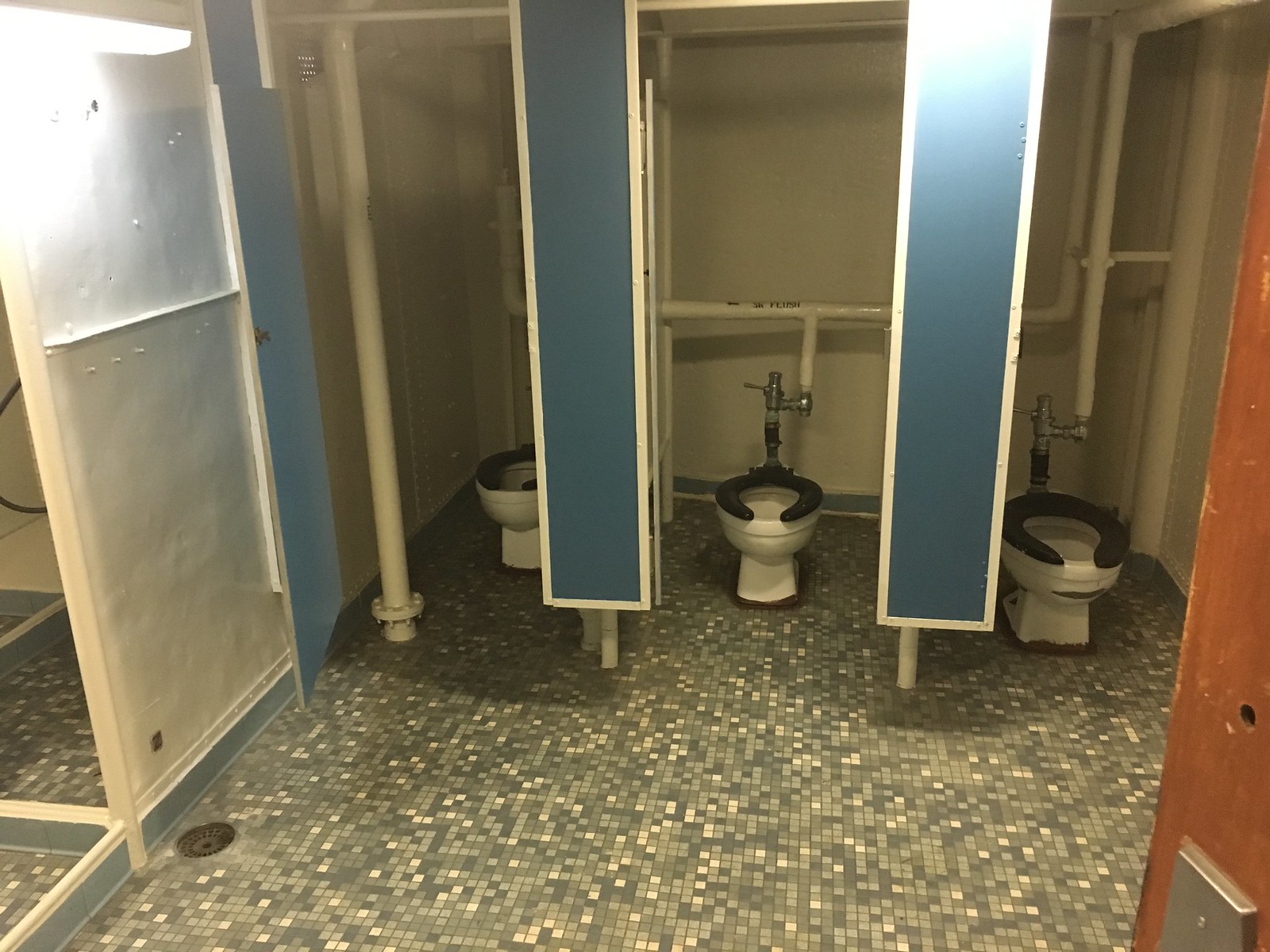This is a detailed photograph of an older public restroom featuring three toilet stalls, each with open blue stall doors. The stalls reveal white toilets with black seats. All toilets are interconnected by visible white PVC piping running along the back. The floor is tiled with a mix of tiny white, gray, and dark gray squares. Visible in the image is a wooden door on the right side, showing signs of wear with scrapes and a small hole, along with a steel kick plate at the bottom. On the left side, there appears to be a glassy door, potentially leading to showers. The walls of the restroom are primarily white, enhancing the slightly worn yet still functional appearance of the space.